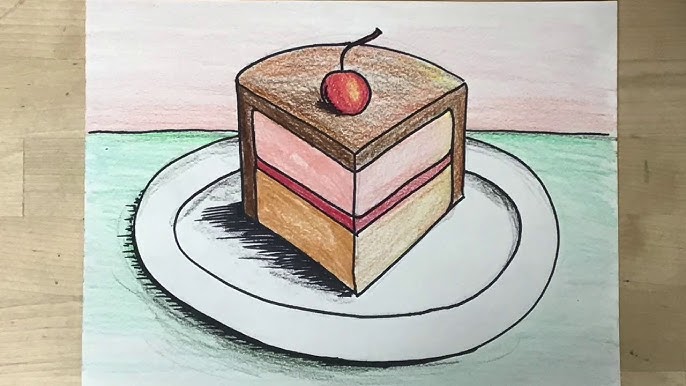This rectangular image captures a photograph of a hand-drawn artwork depicting a delicious slice of pie on a white plate. The drawing is on a piece of paper, placed against a background of light-colored wooden planks with horizontal lines. The pie itself is rendered with meticulous detail: it has a brown bottom layer, a dark red middle layer, and a pink top layer, crowned with a thin chocolate glaze and a bright red cherry with a black stem pointing to the right. The white plate is slightly misshapen and set on a green table, which sits atop a pink background. The paper transitions from white at the top to pink, divided by a black horizontal line, seamlessly blending into the green. This drawing exudes a playful yet realistic charm, vividly capturing the slice of pie and its surroundings.